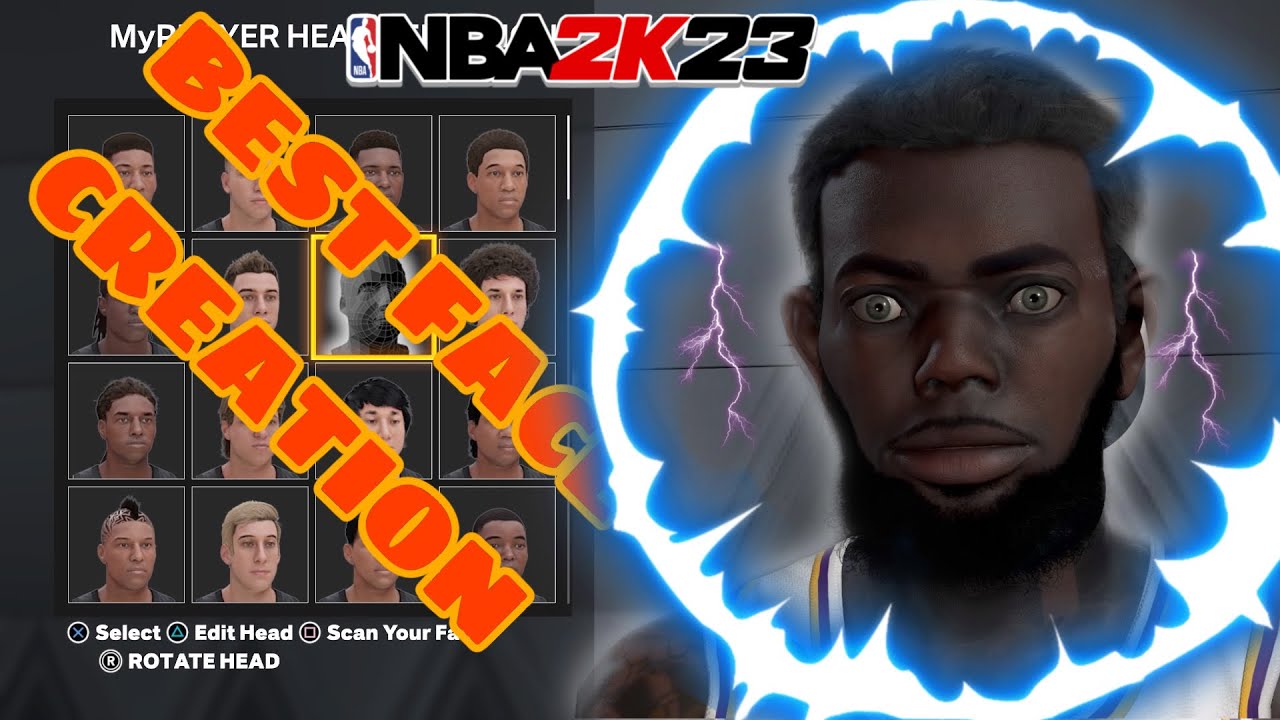A detailed and descriptive caption for the image might be:

"In this vividly detailed screenshot from the player creation screen of NBA 2K23, a 4x4 grid showcases various player avatars that can be customized. The interface includes options to select (X), edit head (triangle), scan your face (square), and rotate head (R). A scroll bar on the right indicates even more customization choices. Overlaid on the screen is the text 'Best Face Creation' in bold, large orange letters, emphasizing the game's robust facial customization feature. The head on the right resembles a blend of Steph Curry and other players, enhanced with a striking blue lightning bolt effect. The interface is unmistakably PlayStation, marked by the classic Sony icons for navigation. This lively scene captures the fun and creativity players can experience in NBA 2K23's diverse and detailed face creation tool."